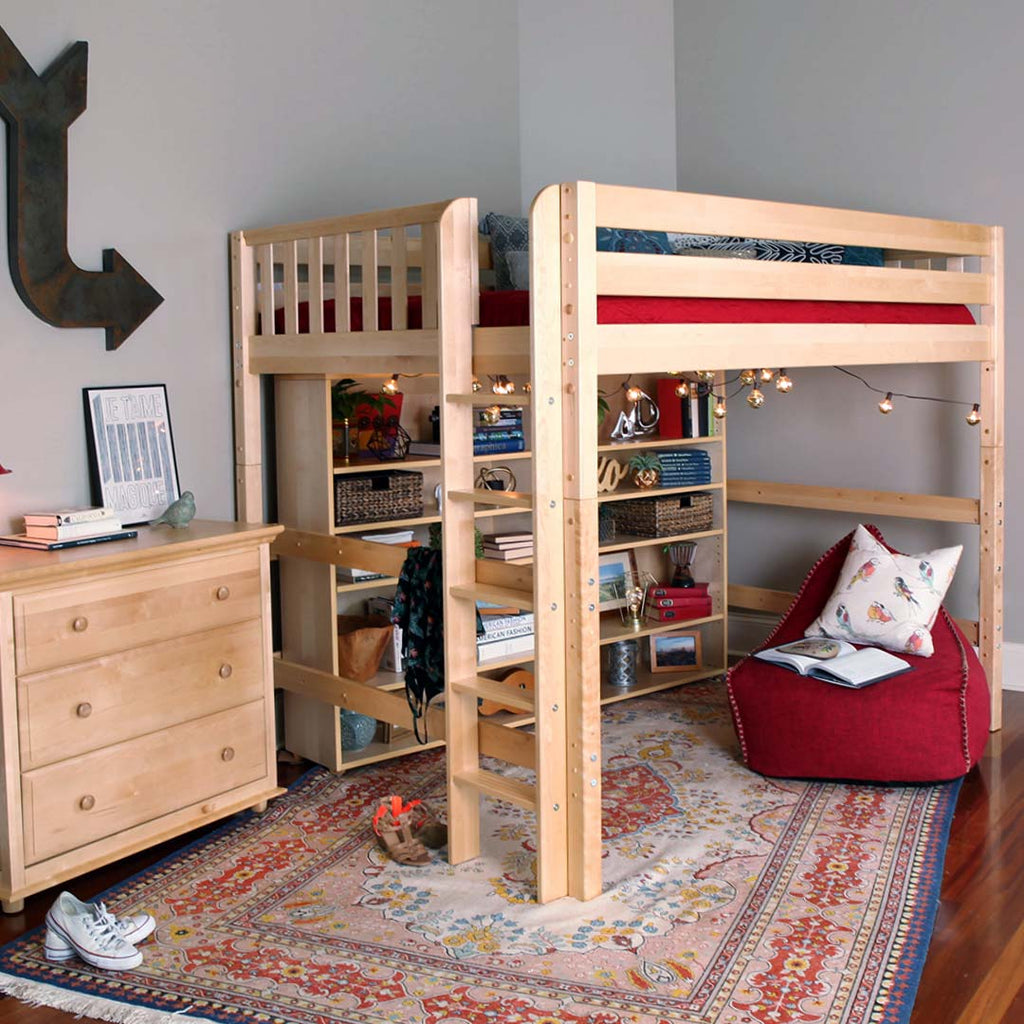The image depicts a child's or preteen's bedroom with muted gray walls and dark wood floors. The centerpiece of the room is a loft-style bunk bed, raised approximately six feet off the ground, accessible by a ladder. Underneath this loft bed is a cozy reading nook featuring a red beanbag chair with a pillow and an open book. Adjacent to the beanbag is a light wood bookshelf stocked with various books and miscellaneous artifacts. The room is decorated with a floral-patterned, multicolored oriental rug in shades of red, pink, blue, white, and yellow.

To the left of the bed is a matching light wood chest of drawers with three drawers. Atop this dresser sits a teal bird figurine, three books, and a piece of monochromatic artwork with the phrase "Je T'aime Magique." The room includes additional details such as a black painted arrow pointing towards the bed and two pairs of shoes on the floor – one pair of white Converses and a brown and orange pair of sandals. The overall atmosphere is warm and inviting, enhanced by decorative lights and a small potted plant under the bed.